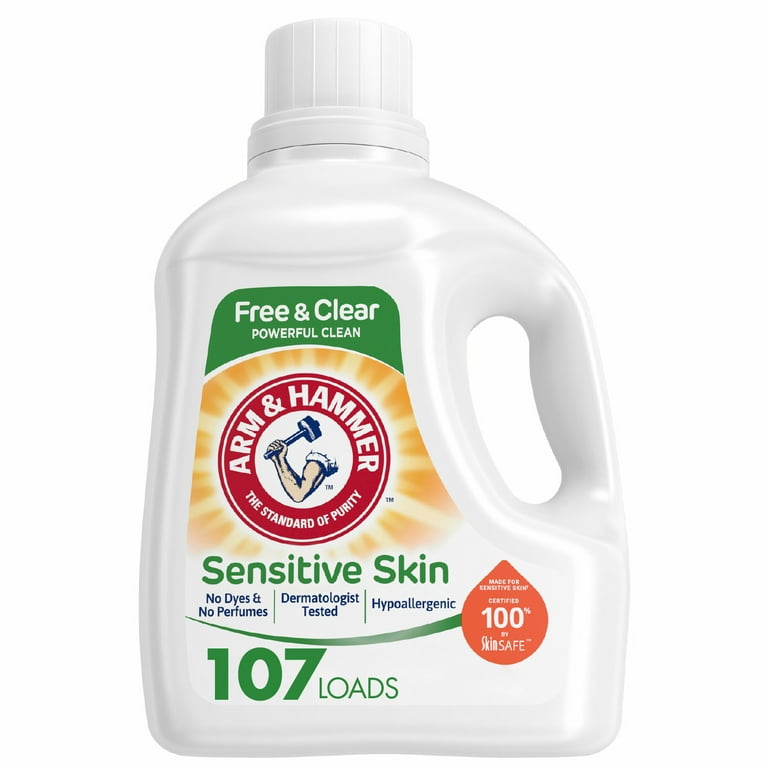The image depicts an Arm & Hammer laundry detergent advertisement, prominently featuring a white plastic jug with a round, grooved cap, suggesting ease of use. The bottle is labeled for "Free and Clear, Powerful Clean" and is specifically formulated for sensitive skin, highlighting attributes like "No Dyes," "No Perfumes," "Dermatologist Tested," "Hypoallergenic," and "Skin Safe." The Arm & Hammer logo is prominently displayed, showcasing a muscular arm wielding a hammer within a red circle, over the declaration "The Standard of Purity." The product is concentrated and capable of handling 107 loads, as indicated twice on the packaging, which also includes a distinctive orange teardrop symbol. The backdrop of the image is stark white, accentuating slight shadows around the jug for a clean and minimalist presentation.